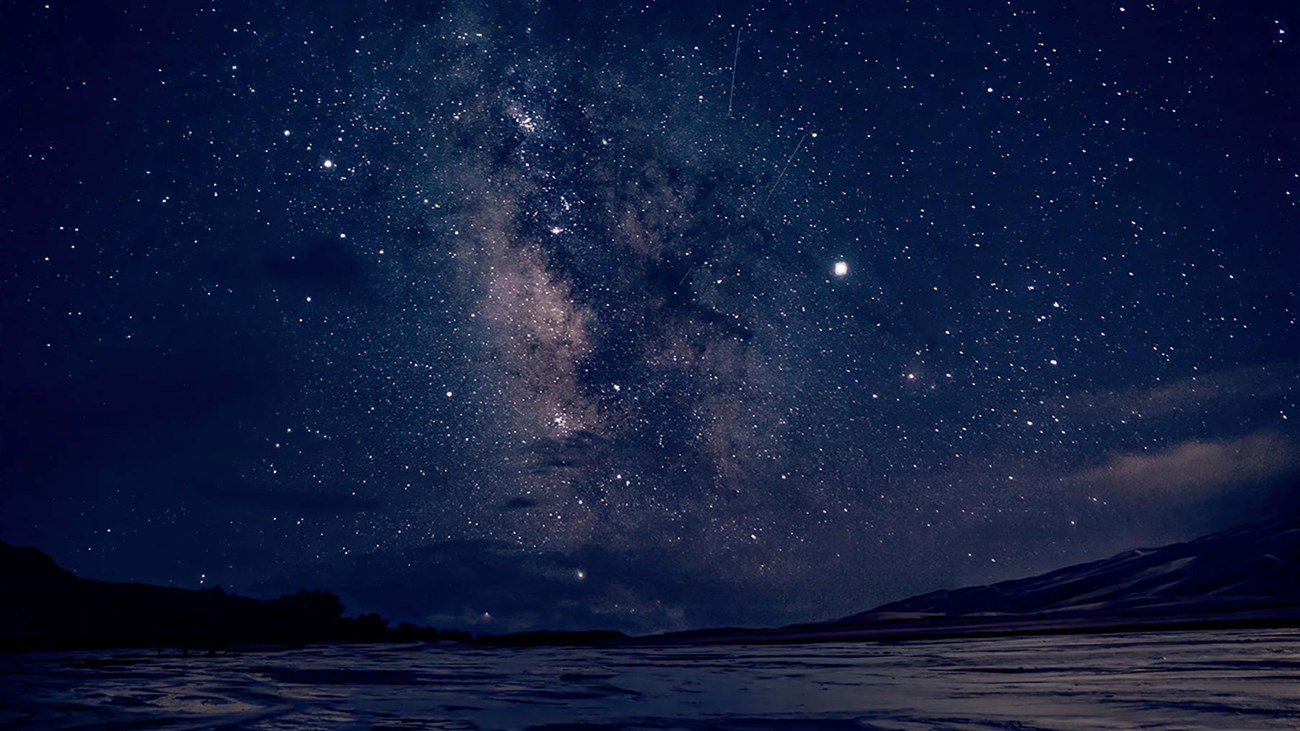This captivating photograph captures a celestial nighttime scene dominated by an expansive, deep navy blue sky, teeming with a million stars of varying brightness and sizes. A striking pink haze stretches down the center of the sky, reminiscent of a cosmic, organic shape indicative of an aurora or nebula. The sky also features misty, cloud-like formations adding to its ethereal beauty. 

Foregrounded is what appears to be either a shimmering body of water or possibly frozen ice, reflecting light in a way that makes it resemble textured desert sand. On the horizon, silhouetted against this magnificent sky, are endless, flat mountain ranges. The mountains are subtle in detail but clear in form, decreasing in height towards the center of the image. Among the stars, one particularly bright star stands out roughly halfway up the sky. 

Overall, the photograph is a mesmerizing blend of celestial charm and barren earth, offering a serene yet awe-inspiring view of the nighttime sky and the silhouetted landscape below.